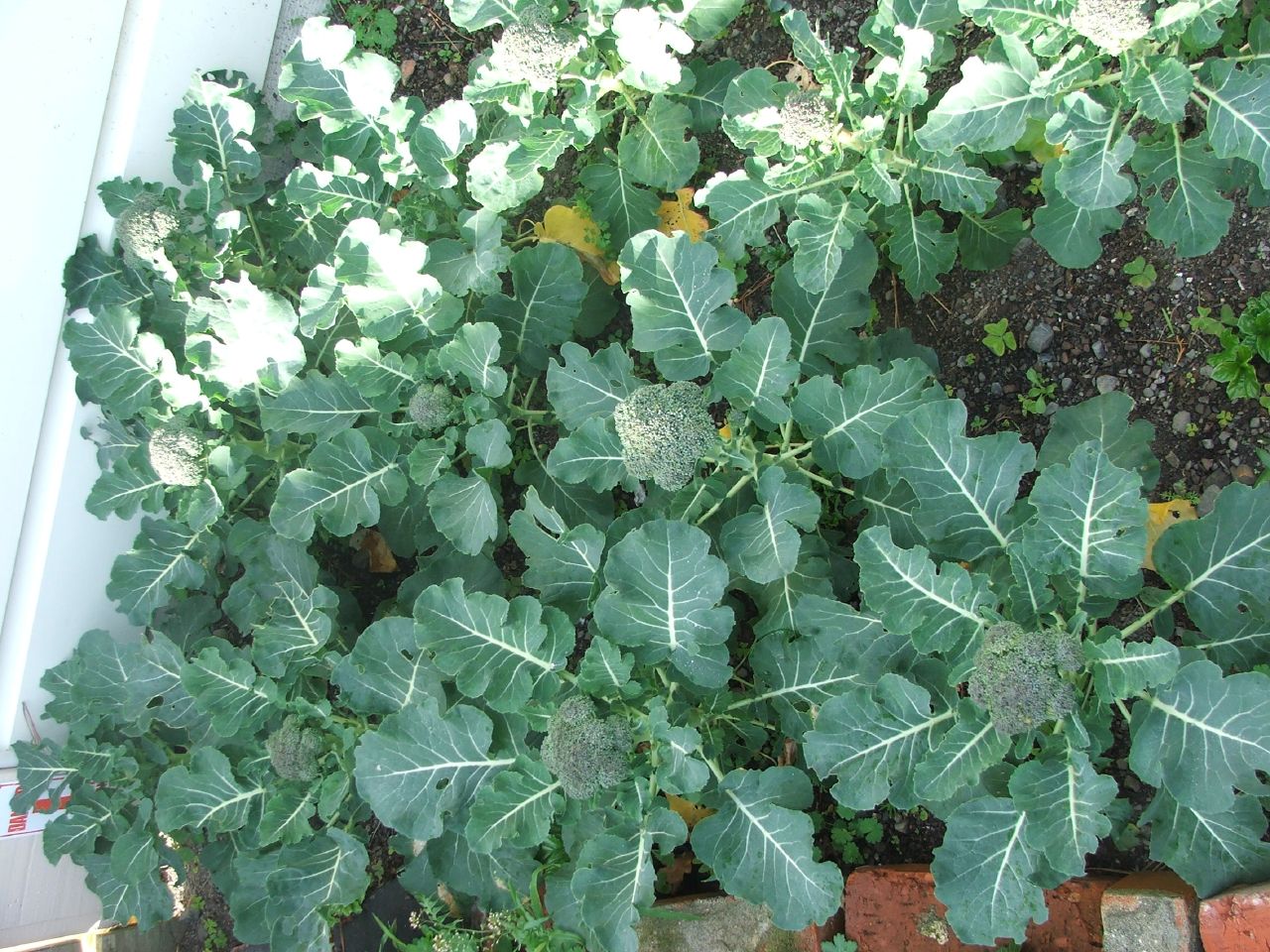This overhead photograph captures a section of a garden bed lined with alternating red and white bricks, situated adjacent to what appears to be the side of a house, identifiable by its shingles on the left. The sun brightly illuminates the top left corner of the image, casting a natural light over the scene. Dominating the garden plot are 10 to 12 vibrant green broccoli plants, each characterized by large, leafy foliage with distinctive thick white veins. The central stem of each plant supports a developing clump of broccoli, varying in size from one plant to another, with hues of green and blue apparent on the mature heads. The dark soil beneath the plants is visible in places, particularly in one relatively empty spot filled with dirt and small pebbles. A white tube is also visible on the left side of the image, adding to the diverse elements captured in this detailed garden scene.